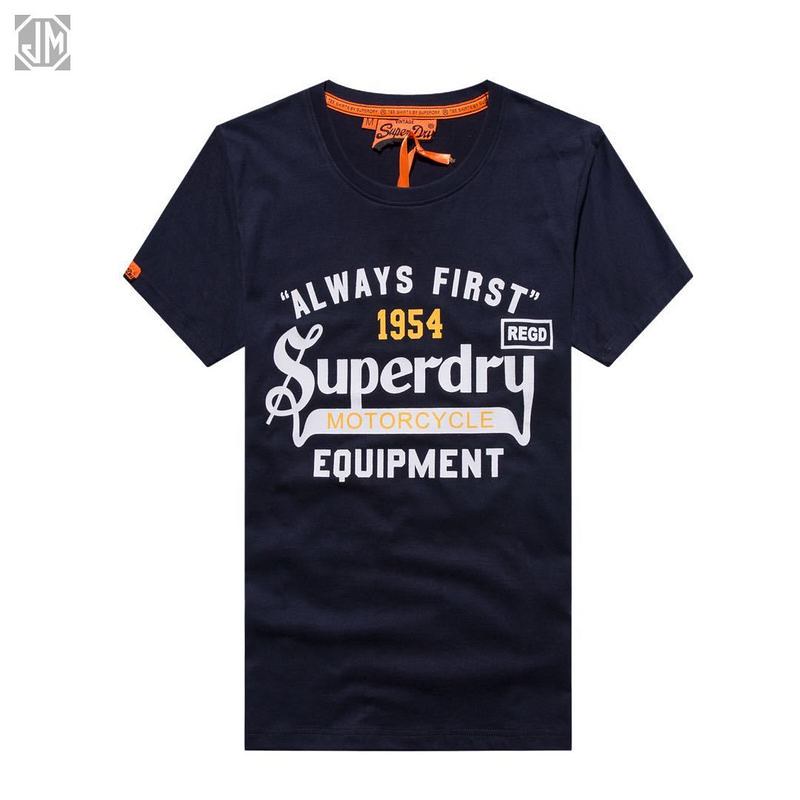The image features a digitally rendered, round-neck, short-sleeved t-shirt centrally positioned against a stark white background, typical of online retail displays. Prominently, in the top left corner, there's a boxed logo with an octagonal outline and the letters "JM" or "KM" in capital letters, showcasing a gray interior. The t-shirt itself is predominantly dark blue or black with an orange interior neck lining and features a visible tag marked "Super Dry," accompanied by an orange ribbon. The shirt is identified as a medium size and bears a green and orange sticker on the right sleeve. At its center, the t-shirt is adorned with bold, creative white text that reads: "Always First." Below this, in yellow letters, "1954" and "Motorcycle" are emphasized. Following this, also in white, is "Super Dry" in the largest, most prominent typeface, with "Motorcycle Equipment" underneath. To the right of "1954," there is a rectangular box with the word "REGD" in capital letters.